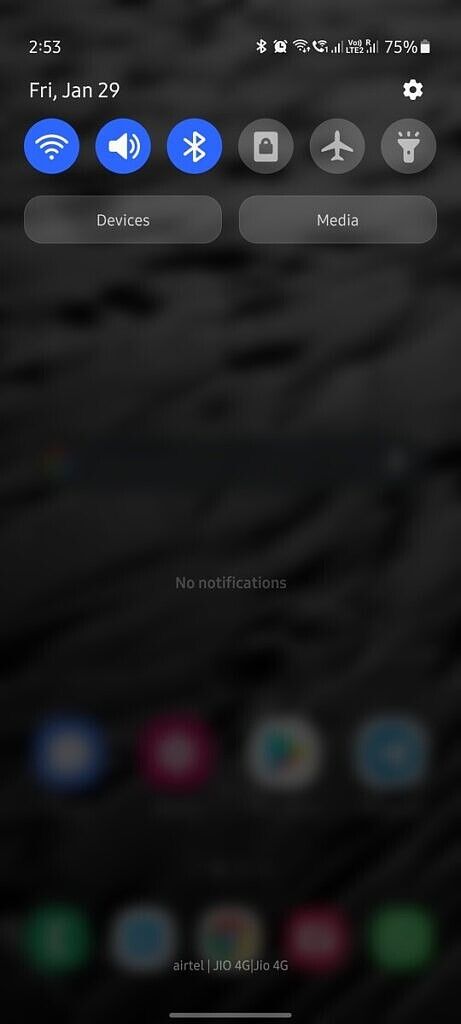This is a mobile screenshot showcasing the quick settings panel on a cell phone's screen. At the top of the panel, various setting icons are visible, including Wi-Fi, sound, Bluetooth, lock, airplane mode, and flashlight. Below these icons, a semi-transparent black button labeled "Devices" with small white text is situated. Adjacent to it on the right, another semi-transparent button labeled "Media" in white text is positioned. In the top right corner, a cogwheel icon indicating further settings is present, while in the top left corner, the date "Friday, January 29th" is displayed. The entire panel is accessed by swiping down from the top of the screen for quick access to these settings, rendering a semi-transparent black filter over the background. Centrally, the text "No notifications" is displayed in small white letters. At the bottom of the screen, blurred images of app icons are faintly visible, with distinguishable icons for Google Play and Facebook Messenger being noted.